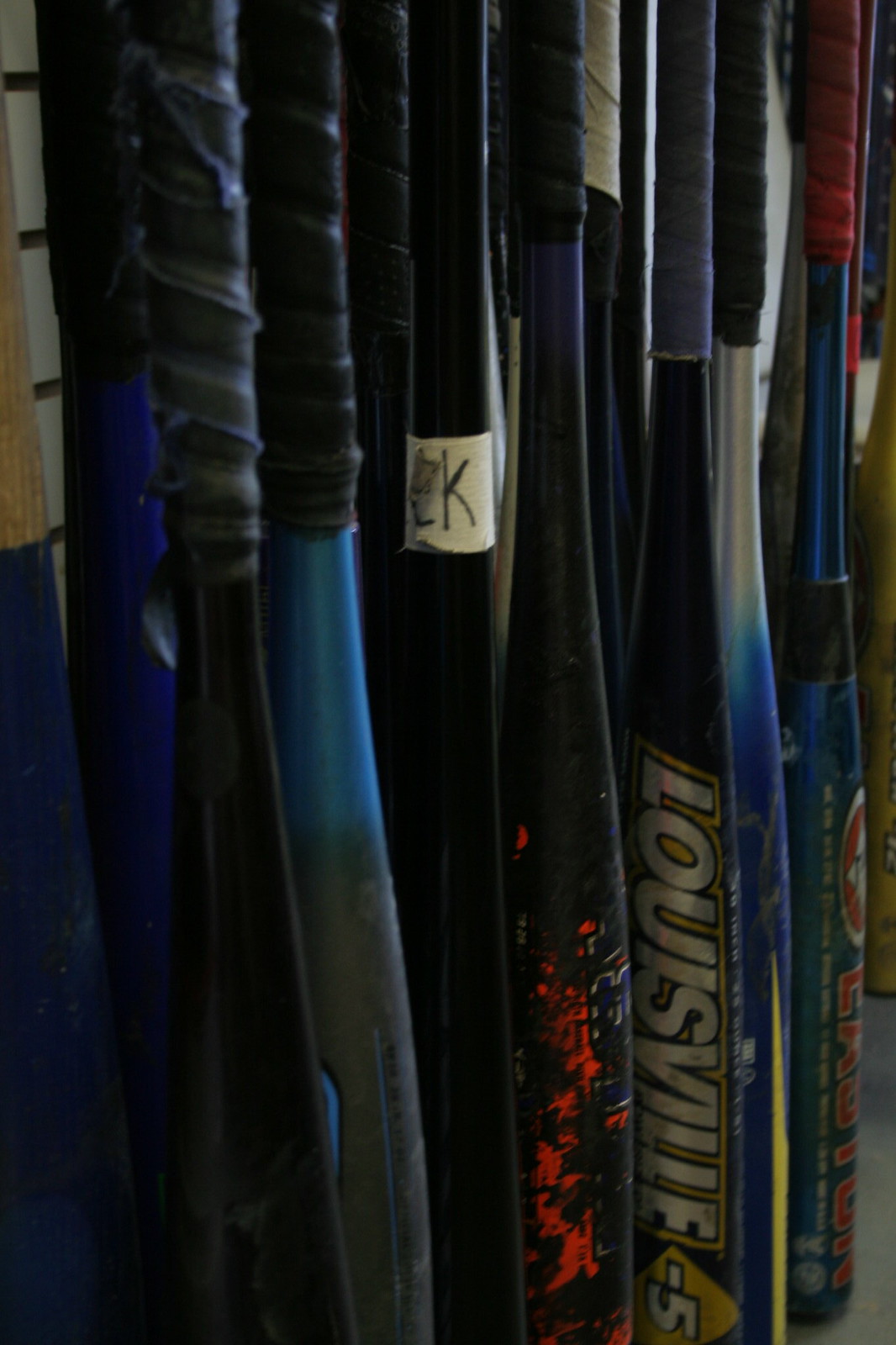This is a slightly out-of-focus, poorly lit, and zoomed-in photograph of the upper handles of a collection of used baseball bats, stacked upright in a room. The photograph does not capture the top or bottom of the bats, preventing a full view. The bats are of various brands and predominantly feature black, blue, and red colors with some bats also showcasing silver accents. The handles, appearing well-worn, are wrapped with different colors of grip tape, including black, red, blue, and white, suggesting they are made of either leather or fabric. One black bat prominently displays "Louisville" in silver letters outlined in black and yellow, while another blue bat seems to have "Eastern" written in red. A baseball bat is also marked with a name tag labeled "CK." Other than these, the bats lack any other visible identifying markers.